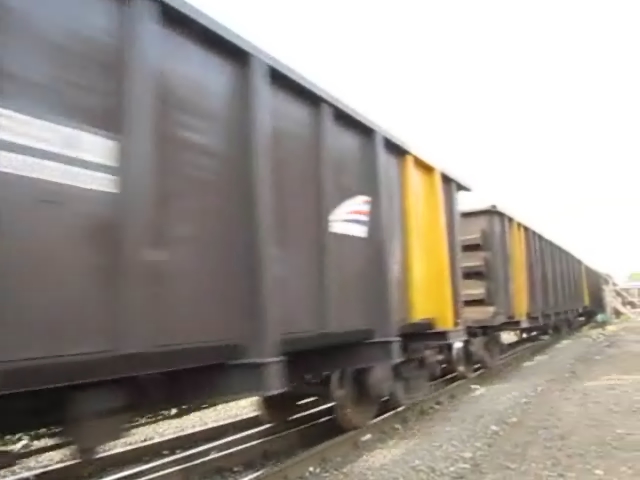The photograph captures a side view of a freight train in motion, evidenced by the blurriness at the forefront of the image. The train travels on a track surrounded by gray gravel, extending into the distance. The train itself is primarily black, featuring a faded white logo with a dark blue line and a red line atop it. The front car exhibits a mix of black paint and bright yellow panels, with additional cars trailing behind. The train wheels and rail appear dark and dirty. Above, a bright, clear sky without clouds beams through, indicating it's a sunny day. In the background, the train moves either toward or away from a distant area with trees and a white structure alongside the tracks. The image also shows a contrast of areas in shade and sunlight, giving a clear indication of afternoon daylight.